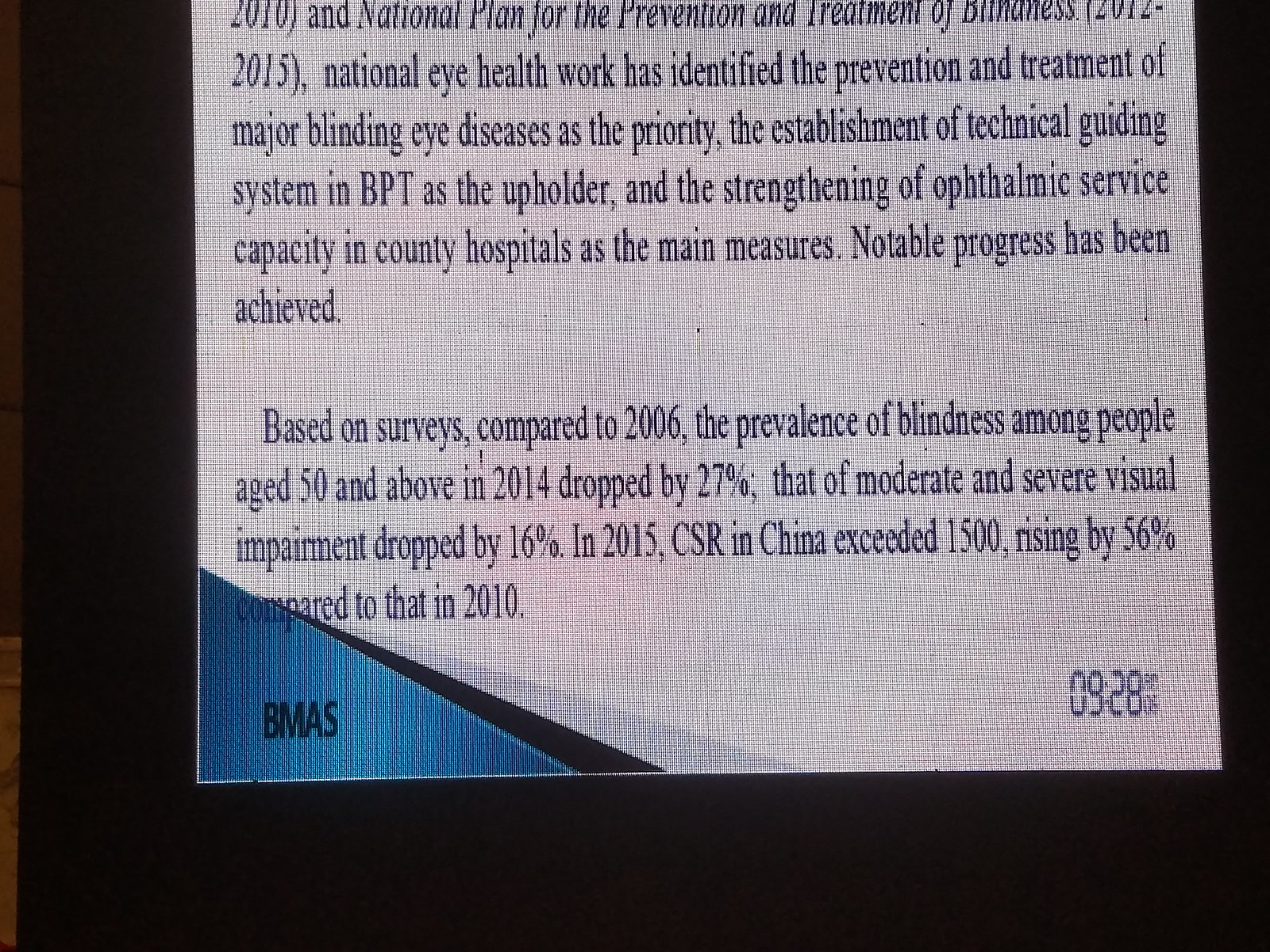The image appears to be a partial screen capture or poster with a black border and a white and gray rectangle containing text. The prominent title reads "National Plan for the Prevention and Treatment of Blindness (2012 to 2015)." The document highlights significant achievements in the field of eye health, specifically emphasizing the identification and treatment of major blinding eye diseases as a priority. Key strategies discussed include the establishment of a technical guiding system, involvement of BPT as an upholder, and enhancement of ophthalmic service capacity in county hospitals. Notable progress is reported: between 2006 and 2014, the prevalence of blindness among individuals aged 50 and above decreased by 27%, while moderate and severe visual impairment decreased by 16%. By 2015, the Cataract Surgical Rate (CSR) in China surpassed 1500, marking a 50% increase compared to 2010. The lower left corner features the acronym "BMAS," while the bottom right corner displays the number "928" or "0928AM."